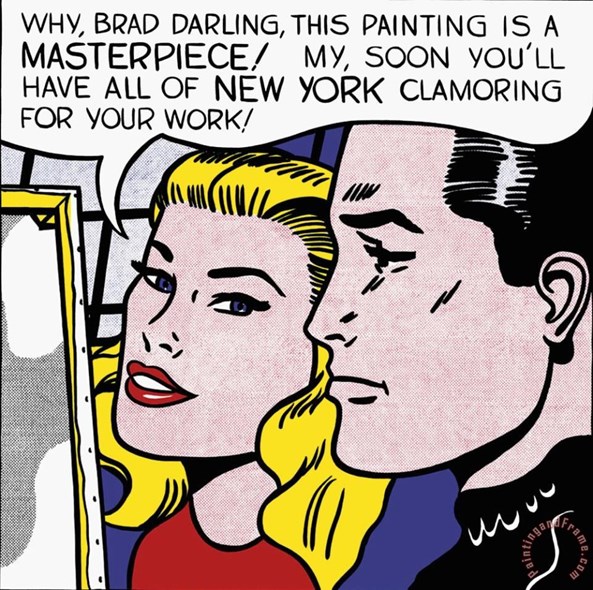The image is a detailed cartoon graphic styled with a dot matrix coloring technique. It prominently features a woman and a man both gazing towards the left, where a white canvas with a yellow frame is placed, its front obscured from our view. A speech bubble emerges from the woman, filled with bold black capitalized text reading, "WHY BRAD DARLING, THIS PAINTING IS A MASTERPIECE. SOON YOU'LL HAVE ALL OF NEW YORK CLAMORING FOR YOUR WORK."

The woman, positioned slightly to the left, has flowing blonde hair, striking blue eyes, red lips, and is adorned in a red top paired with a blue scarf. The man, to the right, sports a black turtleneck, short black hair, and subtle white accents on his shirt resembling inverted curves. The background showcases a black window frame inset with blue glass. Additionally, the bottom right corner of the artwork bears the logo "painting and frame.com."